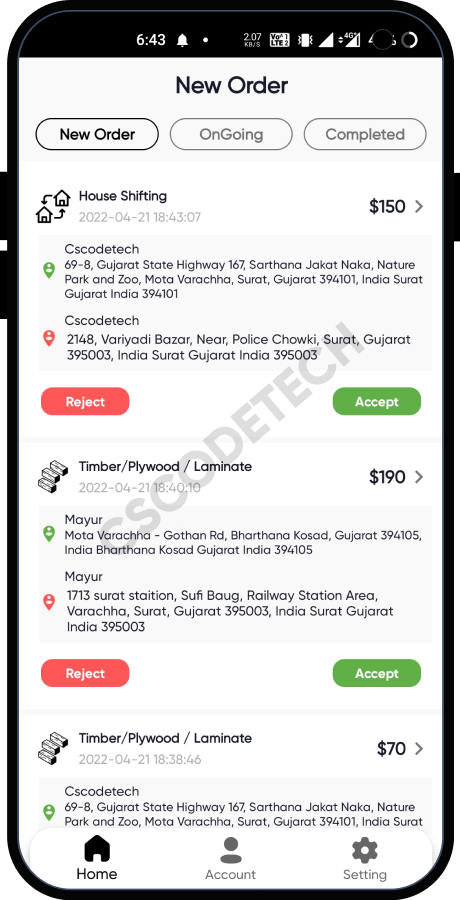### Detailed Screenshot Description:

The screenshot depicts a smartphone interface with several key elements, primarily showcasing a new orders management screen. 

- **Top Bar Elements:**
  - **Timestamp:** "06:43"
  - **Icons:**
    - A notifications bell
    - Camera icon
    - Data speed indicator displaying "247 KB/s"
    - LTE signal indicator
    - Wi-Fi signal icon
    - Battery icon

- **Main Screen:**
  - **Header:** "New Order" in white text over a black background.
  - **Tabs:** There are three tabs labeled "New Order," "Ongoing," and "Completed." The "New Order" tab is currently selected.
  
  - **First Order:**
    - **Shipping Address and Timestamp:**
      - House icon
      - "Shipping 22/04/21" timestamp "18:43:07"
    - **Order Amount:** "$150"
    - **Navigation Arrow:** Right-facing arrow
    - **Order Details:**
      - Text reading "CSCODTECH, 698 Gujara (Gujarat State Highway 161, Sothania to Tarka Naka, Nature Park Zoo, Motovracha, Surat, Gujarat 394101, India. Surat, Gujarat, India 394102)."
    - **Action Buttons:** "Reject" (red) and "Accept" (green)
    - **Watermark:** "CSCODTECH"
  
  - **Second Order:**
    - **Product Types:** "Timber / Plywood / Laminate"
    - **Order Amount:** "$190"
    - **Navigation Arrow:** Right-facing arrow
    - **Shipping Timestamp:** "22/04/21" timestamp "18:40:10"
    - **Action Buttons:** "Reject" (red) and "Accept" (green)
  
  - **Third Order:**
    - **Product Types:** "Timber / Plywood / Laminate"
    - **Shipping Timestamp:** "22/04/21" timestamp "18:38:46"
    - **Order Amount:** "$70"
    - **Action Buttons:** "Reject" (red) and "Accept" (green)

- **Bottom Navigation Bar:**
  - Three icons are present:
    - Home icon
    - Account icon
    - Settings icon

This detailed caption captures all critical visual and textual elements within the given smartphone screenshot, providing a clear and comprehensive description.